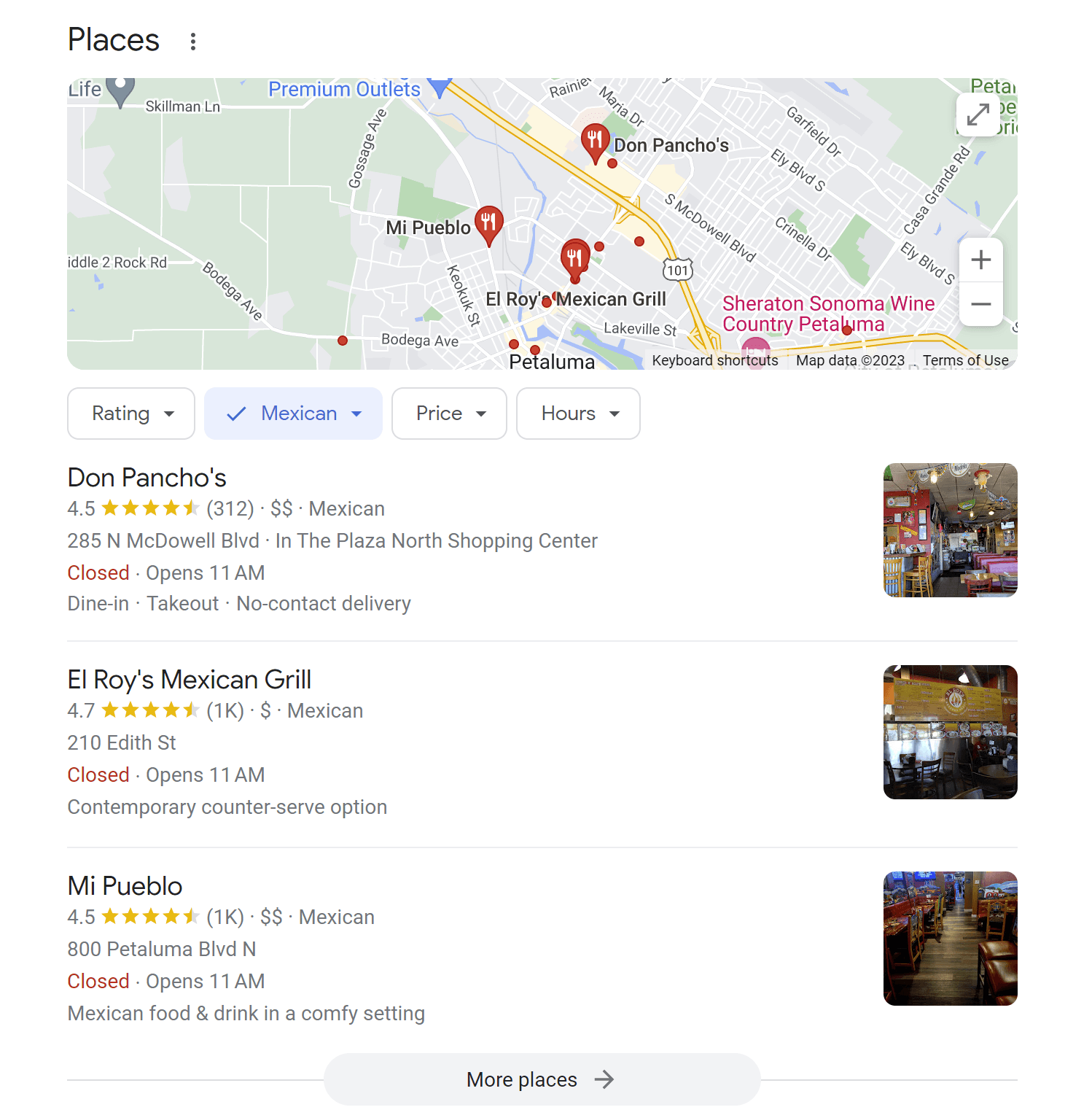The image displays a Google search result for local Mexican restaurants. At the top, the header "Places" is visible, followed by a map highlighting the locations of three specific eateries marked with red icons featuring a fork and knife. The roads S. McDowell Boulevard, Garfield Drive, and Bodega Avenue are also visible, with a prominent yellow road indicating a main thoroughfare.

Below the map are three listings: 
1. **Don Pancho's** - Located at the top of the list.
2. **El Roy's Mexican Grill** - Positioned as the second entry.
3. **Mi Pueblo** - Listed in the third spot.

Each listing includes a detailed breakdown featuring:
- The star rating of the restaurant.
- A classification as a Mexican restaurant.
- Price range indicators.
- The address and hours of operation, with a note that all are currently closed.

Additionally, there is a brief description provided for each establishment, summarizing the type of food and drink they offer.